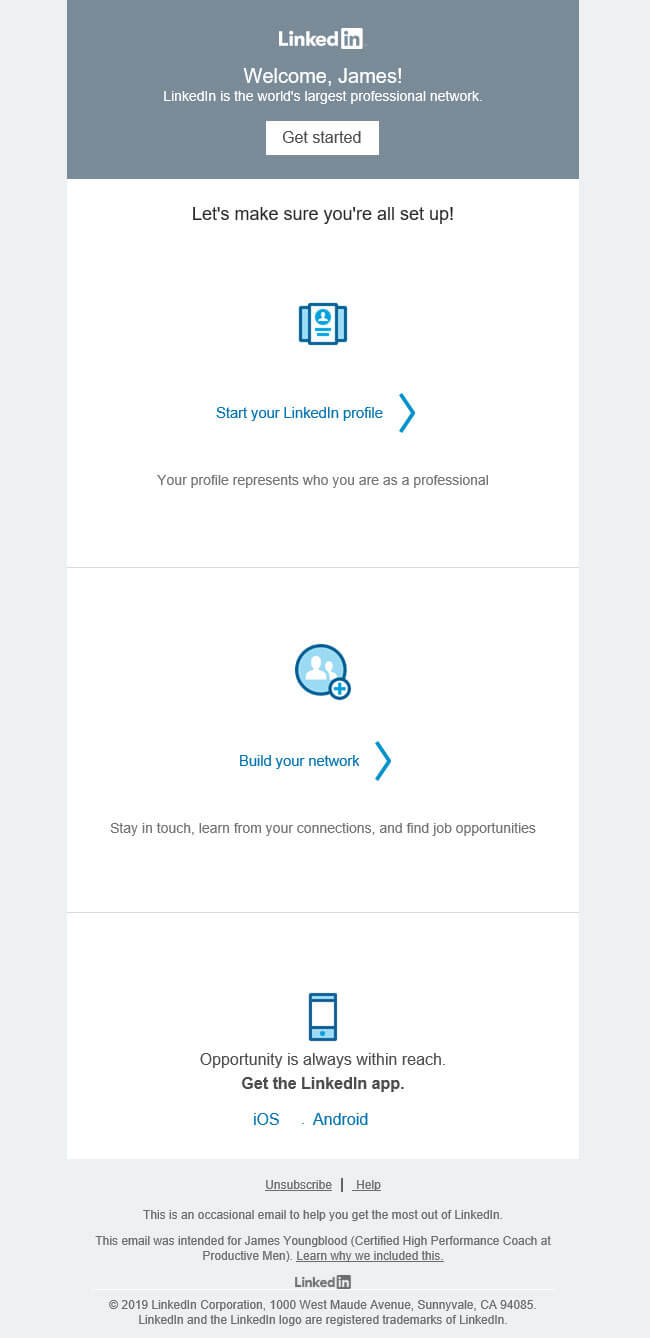A detailed screenshot is captured from a phone or a web page, formatted as a tall rectangle. The background is predominantly off-white and light gray. At the very top of the image, there is a gray rectangle with the LinkedIn logo in white lettering, accompanied by the text "Welcome James". Below, a brief description states, "LinkedIn is the world's largest professional network". This section also features a prominent white button with gray text that reads "Get Started".

The body of the web page is primarily white with gray and blue accents. The main heading in gray reads, "Let's Make Sure You're All Set Up". Below the heading, there is a blue link that says, "Start Your LinkedIn Profile", accompanied by a blue arrow pointing to the right. Another blue link, "Build Your Network", is also present with a corresponding blue arrow. Subtext in gray states, "Stay In Touch, Learn From Your Connections, and Find Job Opportunities".

Towards the lower part of the image, there's a section promoting the LinkedIn mobile app. This includes the text, "Get the LinkedIn App," followed by links for iOS and Android. The links are visually distinguished and encourage users to download the app for their respective devices.